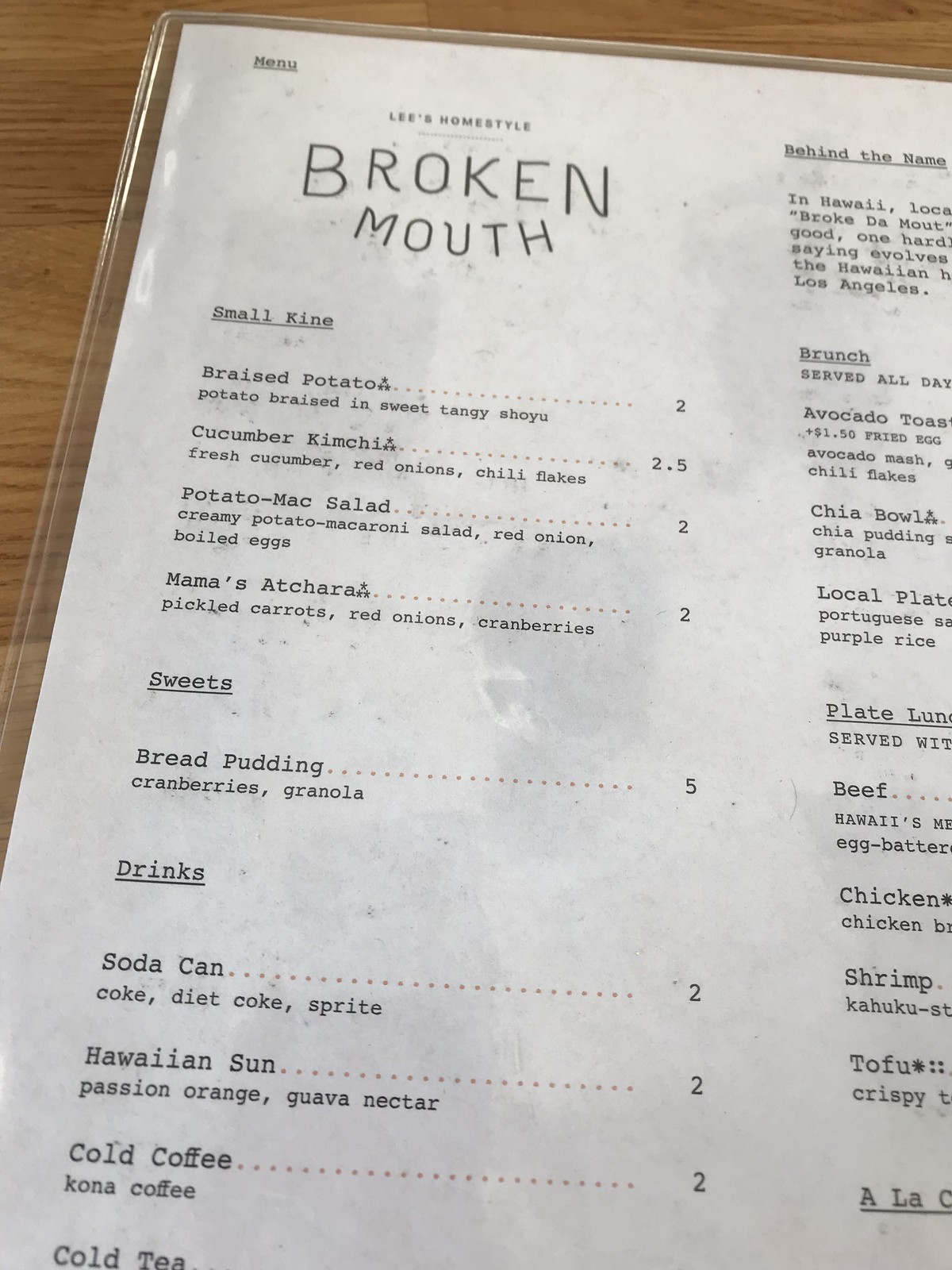This photograph captures the top left corner of a restaurant menu from "Lee's Homestyle Broken Mouth." The menu is printed on white paper that shows a faint texture or pattern, possibly indicating wear or lack of cleanliness, and it is encased in a clear plastic sleeve. The menu rests on a light tan-colored wooden table. The text is presented in a black, serif typewriter-style font.

At the top left, the word "Menu" is underlined, followed by the restaurant's name, "Lee's Homestyle Broken Mouth." Below that, different sections of the menu are listed, starting with "Small Kind." This section includes items such as:

- Braised Potatoes: Potato braised in sweet tangy shoyu - $2
- Cucumber Kimchi: Fresh cucumber, red onions, chili flakes - $2.50
- Potato Mac Salad: Creamy potato-macaroni salad, red onion, boiled eggs - $2
- Mama's Atchara: Pickled carrots, red onions, cranberries - $2

Following the "Small Kind" section is the "Sweets" section, which is underlined and features:

- Bread Pudding: Cranberries, granola - $5

Next, the "Drinks" section lists various beverages:

- Soda Can: Coke, Diet Coke, Sprite - $2
- Hawaii Sun: Passion Orange, Guava Nectar - $2
- Cold Coffee: Kona coffee - $2
- Cool Tea - (specifics not mentioned)

At the top of the menu, a brief description about the restaurant's name is partially visible, but cut off. Additional sections, such as "Brunch" and "Plate Lunch," are mentioned but are obscured as they extend beyond the edge of the photographed area.